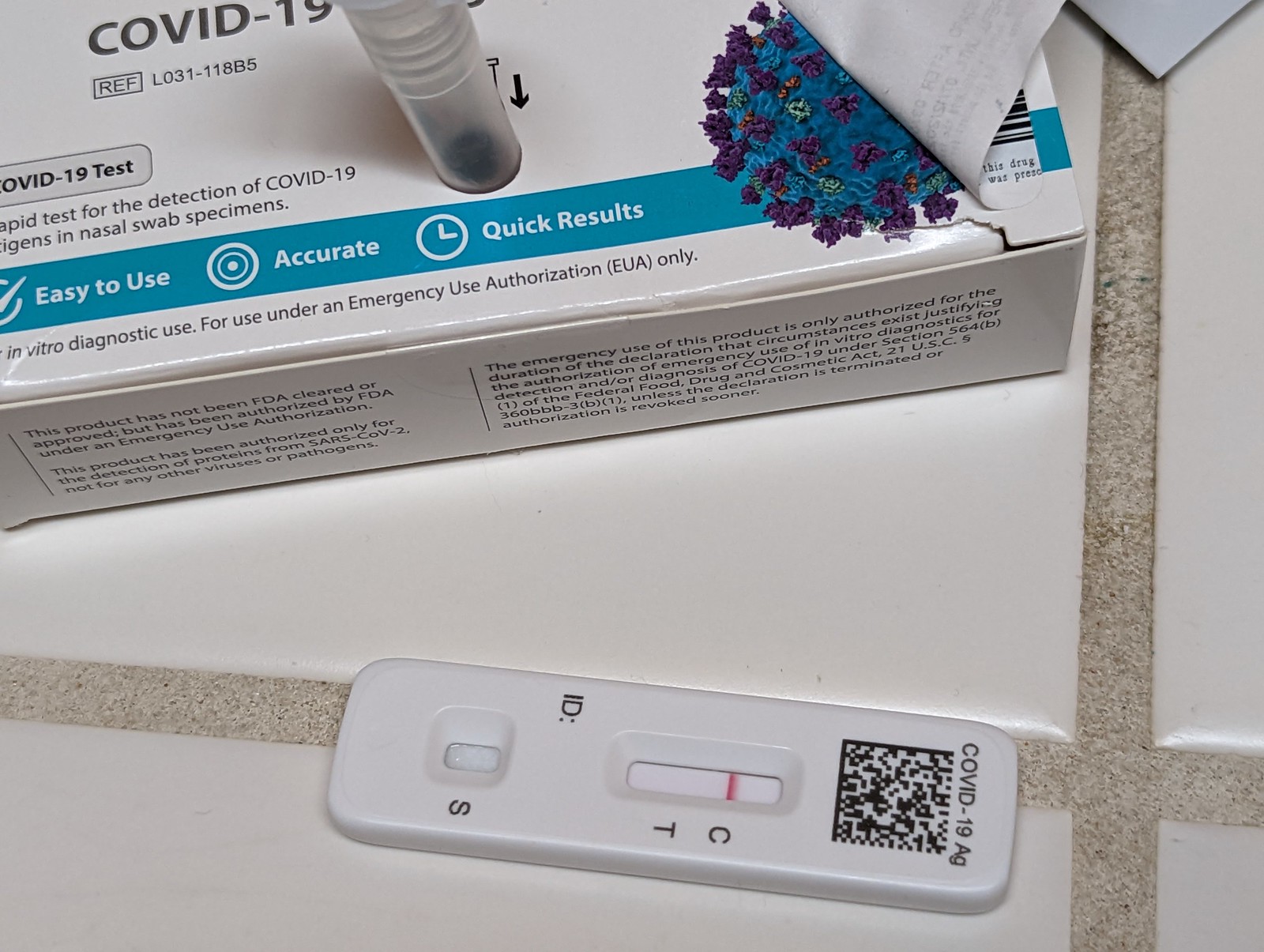The image depicts a COVID-19 test kit nestled within an open box. The box is placed on a ceramic-tiled floor, evident from the bottom half and bottom right sections of the image. The floor tiles are square-shaped and predominantly white. Their divisions are marked by grout lines that appear to have a rough granite texture, varying in shades of light brown and dark gray.

At the bottom of the image lies a rectangular COVID-19 test device. The top of the device prominently displays the term "COVID-19 AG" along with a square QR code just below it. In the middle section of the device, there is a rectangular window with a white background featuring a red line. To the right of this window are the letters "C" and "T," vertically aligned, with additional letters "ID" and "S" positioned at different points on the device.

The top half of the image showcases a larger box with the label "COVID-19 RDF COVID-19 test." Additional text on the box mentions that the kit is "easy to use," "accurate," and provides "quick results" in white font against a bluish-teal background. The box also includes some clear plastic tubing, readily observable.